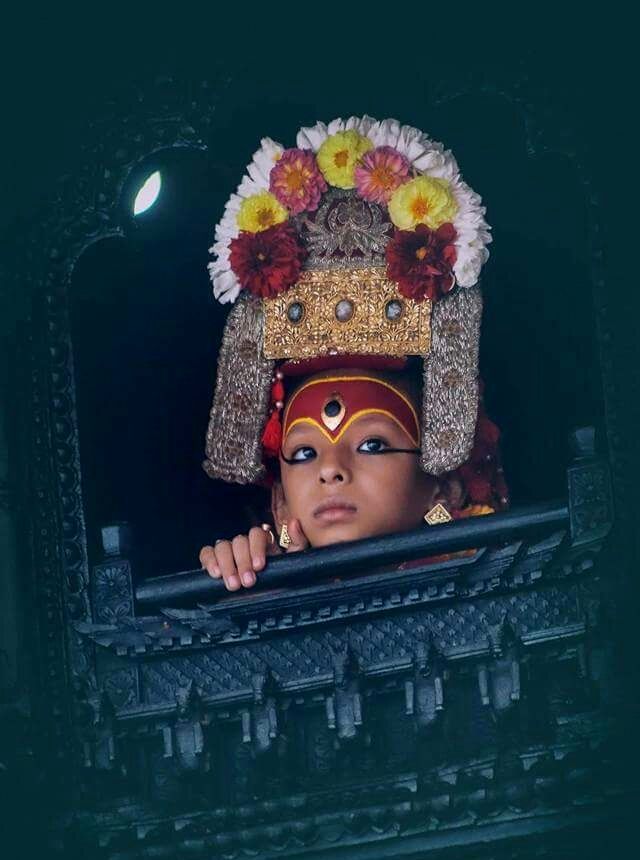This vertically oriented photograph captures a child, possibly of Asian descent, peering through an elaborate, ornamental window frame. The entire frame is black and highly detailed, adorned with carvings and intricate patterns including a row of six carved horse figures. The child's face is the focal point, enhanced by dramatic makeup; their under-eyes are heavily lined with eyeliner extending towards their ears, and their forehead is painted red with a yellow outline, topped with a central golden jewel featuring a black center. Their expression is neutral, and they are looking slightly up and to their left.

The child's headdress is striking and tall, composed of a golden rectangular section adorned with three horizontal stones. Above this, a crown of vibrant flowers in white, blue, pink, yellow, and red rests. The headdress features two ornamental fabric pieces hanging down either side of the face, supported by highly decorated steel supports. Additionally, they wear large gold earrings. The detailed wooden frame is accentuated by light shining from the upper left, adding a dramatic highlight to the scene, with the child's hand visible as they rest it on the edge of the ornate window.